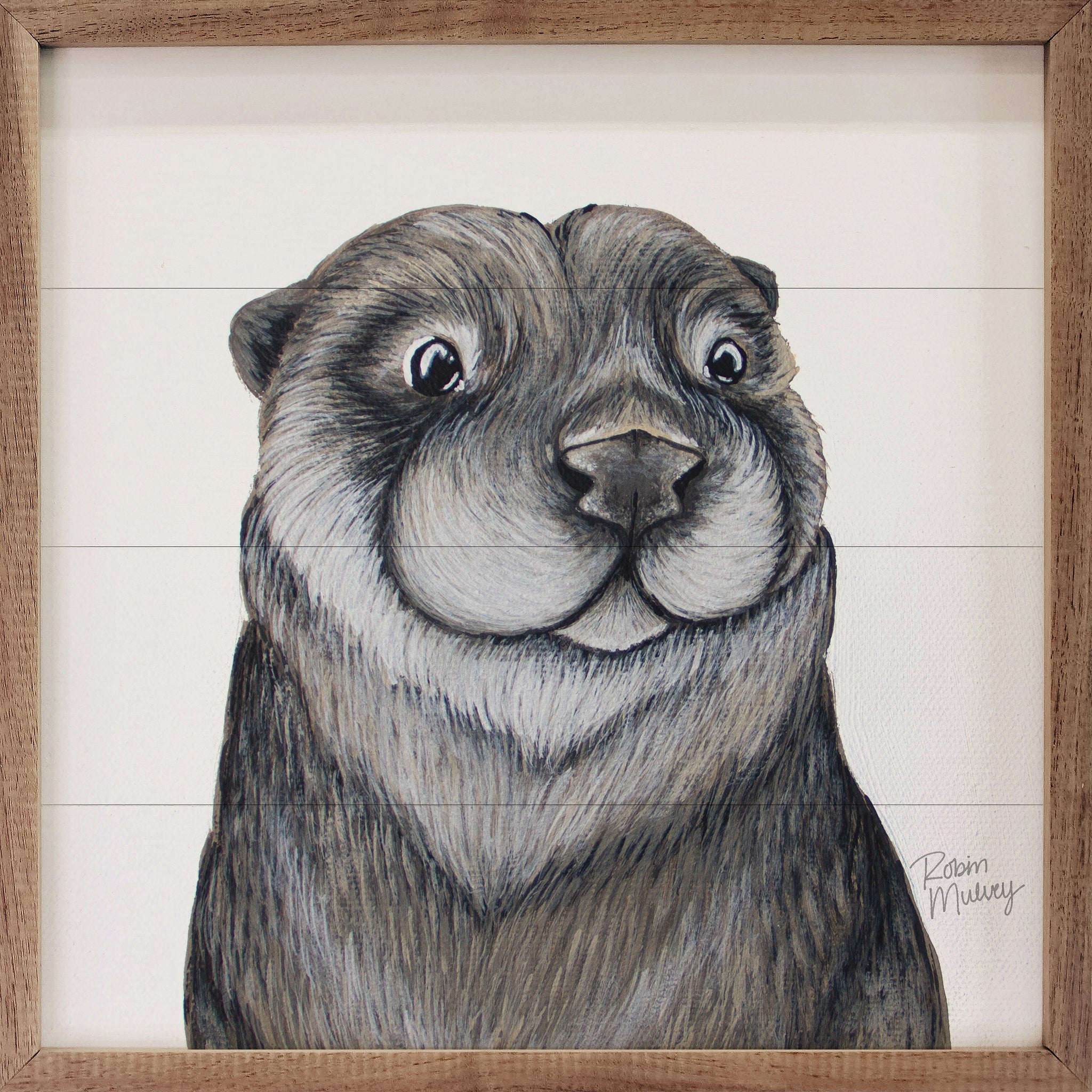The image is a highly detailed painting of an otter, set against a cream-colored background and framed in a brown wooden frame. The otter's fur, exquisitely rendered with either charcoal-like pencils or a very fine brush, displays a rich variety of colors ranging from darker shades to lighter ones, with white fur interspersed. The otter has a distinctive white beard and a well-defined nose. Its black, shiny eyes stand out prominently, giving it a lifelike appearance. The fur around its face forms a circular pattern, and its small, pointed ears extend to either side. The lower right-hand corner of the artwork features the signature of Robin Mulvey. Additionally, three horizontal lines subtly cross the painting, adding an artistic dimension to the detailed portrayal of the cute and chubby-looking otter.